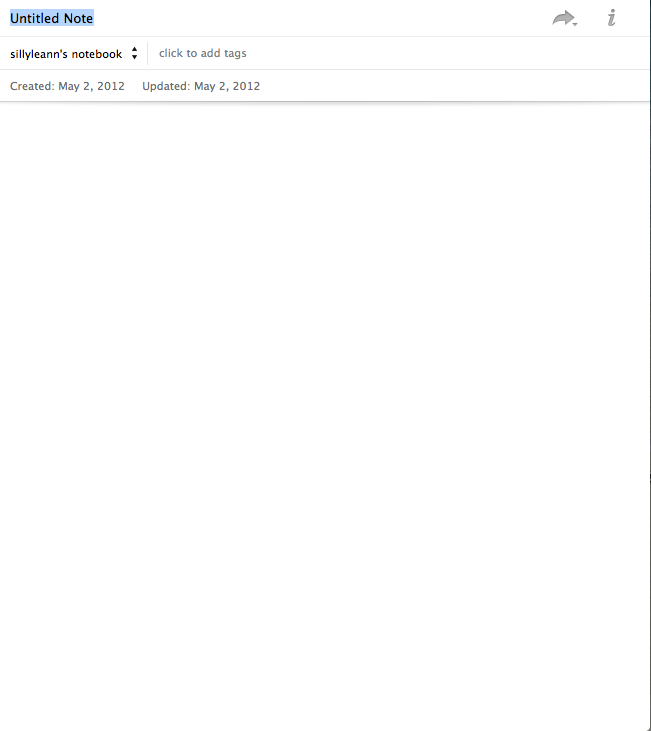The screenshot depicts the interface of a note-taking application with a prominently empty white space occupying the majority of the screen. At the top of the interface, there is a highlighted text field labeled "Untitled Note," indicating that the title is likely being edited by the user. Just below this field, the text "Silly Leanne's Notebook" suggests that the note belongs to a notebook named by a user named Leanne, who whimsically refers to herself as "Silly Leanne."

Adjacent to the notebook title, there is an option labeled "Click to Add Tags," allowing the user to categorize the note with tags. Below these elements, the note's creation and last update dates are displayed, both marked as May 2, 2012. Additionally, the top of the screen features a right-facing arrow icon, which likely functions as a send button, and an eye icon, presumably for accessing more information.

The overall interface appears minimalistic, with no other visible content or additional notes, highlighting an almost entirely white space that underscores the lack of additional information or entries in the note.